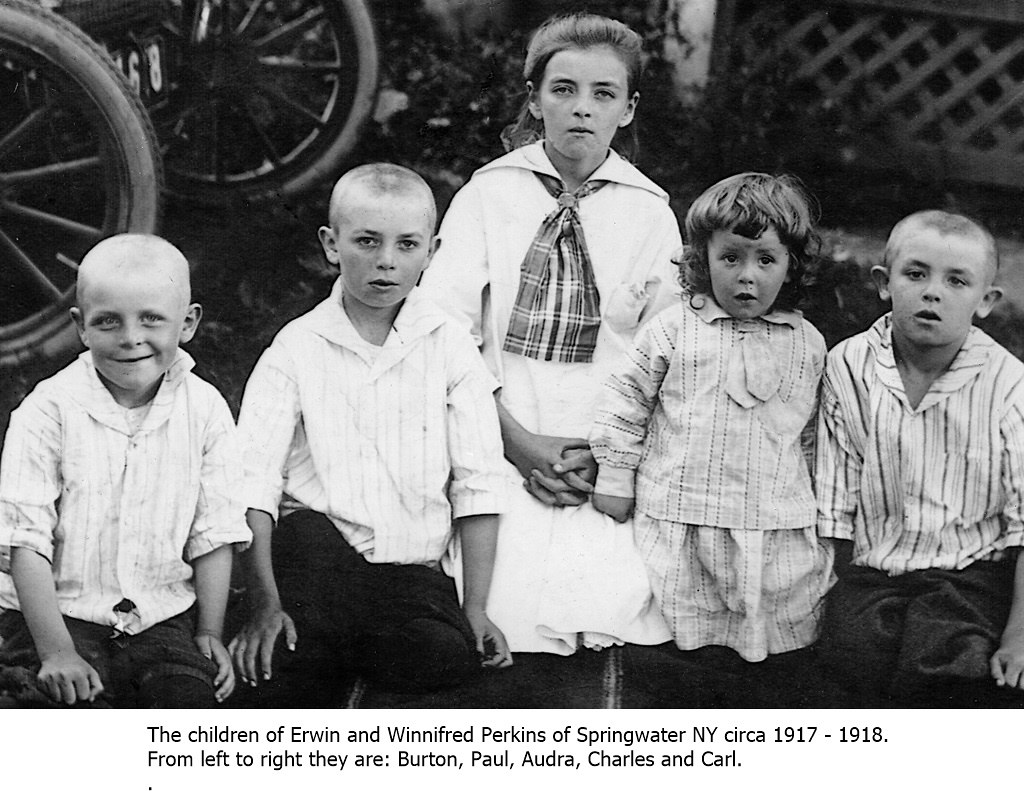In this black-and-white photograph dated circa 1917 to 1918, five children are seated together in front of a background that includes a building, a fence, and two partially visible objects with wheels, possibly old cars or motorbikes. From left to right, these children are identified as Burton, Paul, Audra, Charles, and Carl, the children of Erwin and Winifred Perkins of Springwater, New York. The boy on the far left, Burton, has a nearly bald head and wears a vertically striped shirt with dark pants. Next to him, Paul sports a buzz cut and larger ears. In the center, the tallest child, Audra, is a girl wearing a scarf around her neck and a white dress. Beside her is a younger girl, Charles, who wears a white dress with some stripes and a bow tie. On the far right, Carl, another boy with a crew cut and larger ears, is dressed similarly in a white and striped shirt with dark pants. The children generally have neutral expressions, with only Burton showing a hint of a smile. The photograph captures a nostalgic and still moment from the early 20th century.